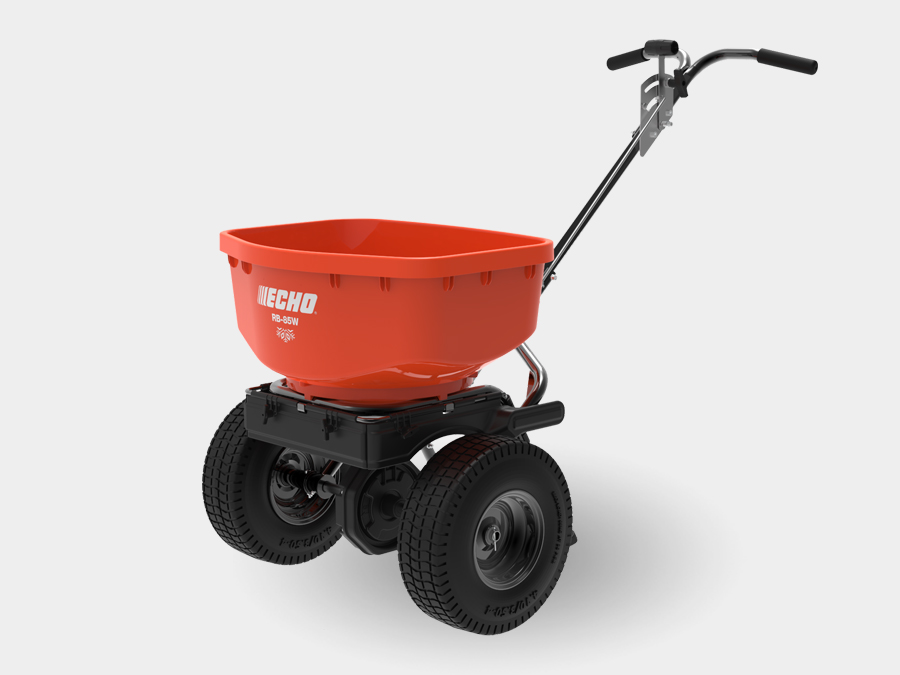The image portrays a lawn seed spreader prominently featuring a red hopper atop a solid black base. This base is equipped with two substantial, wide tires with grayish rims, ensuring stability and mobility. Stemming from the base is a silver aluminum handlebar, branching out at the top into two grips akin to bicycle handlebars, designed for ergonomic handling. Attached to this handlebar is a switch lever, likely for regulating the seed dispersal rate or halting the distribution when needed. The spreader bears the brand name "ECHO" clearly on its red portion, potentially indicating its manufacturer. Additionally, there is a partially obscured model number, R-8-5-W, that adds to its detailed specifications. The red part appears to be made of lightweight metal or hard plastic. The entire setup is presented against a stark white background, emphasizing the product's functionality and design, which could mistakenly suggest it as a utility cart or bucket for carrying various items.